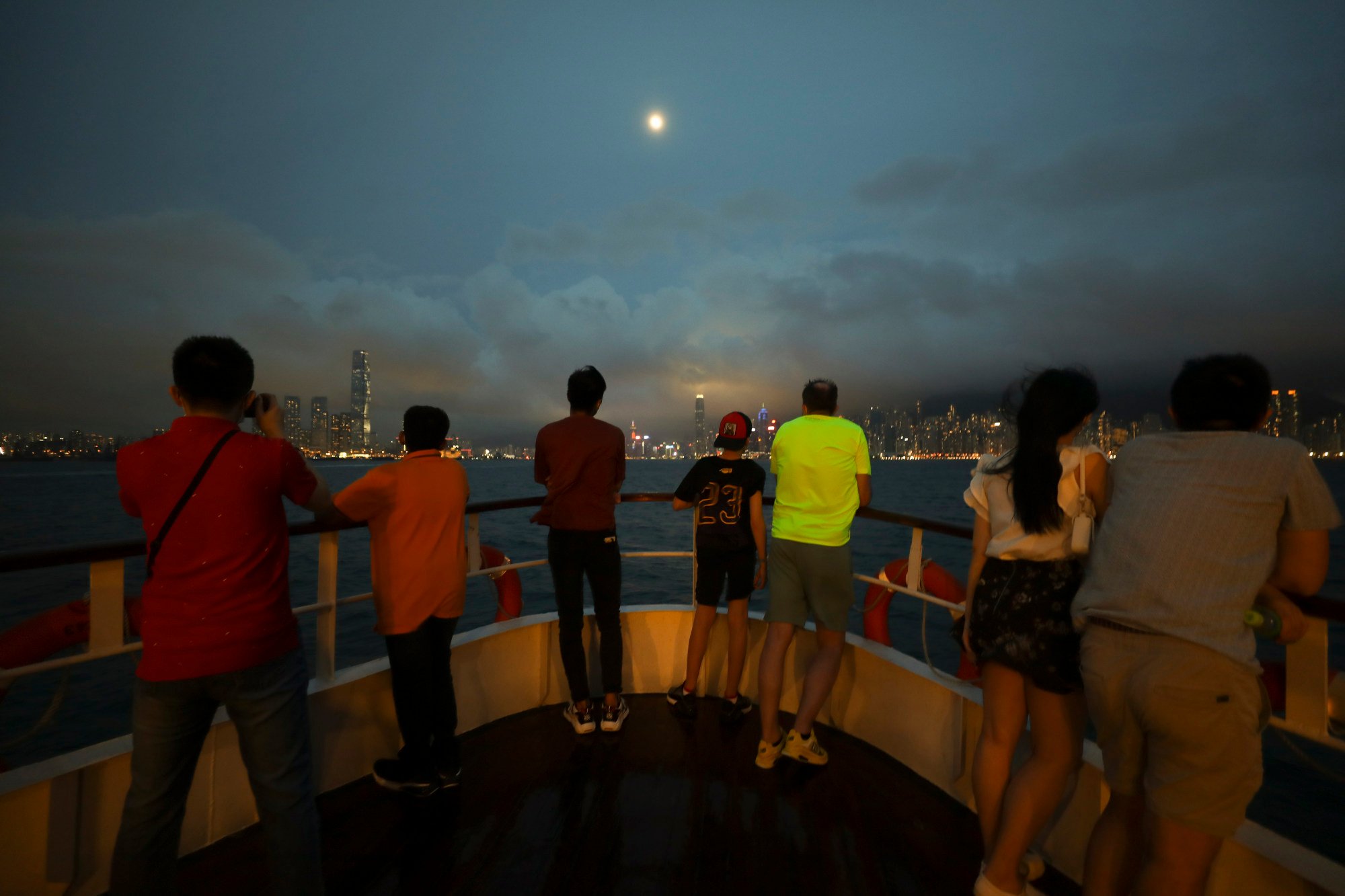A group of seven people stands at the bow of a sightseeing boat, dressed casually and gazing intently towards a modern, illuminated city skyline. The boat's deck has dark wood and a curved railing adorned with red life rings, emphasizing the nautical atmosphere. The scene is set at night under a high, full moon, which illuminates the thick cloud cover above the city's numerous lit-up skyscrapers. One man with short black hair, wearing a red polo shirt and jeans, is captured in the moment of photographing the stunning cityscape. Another man, standing beside him in an orange polo shirt and jeans, also looks towards the horizon. The boat floats on dark blue water, creating a serene yet vibrant backdrop against the vast sky transitioning from light blue at the horizon to darker shades as it extends outward, highlighting the picturesque beauty of the moment.